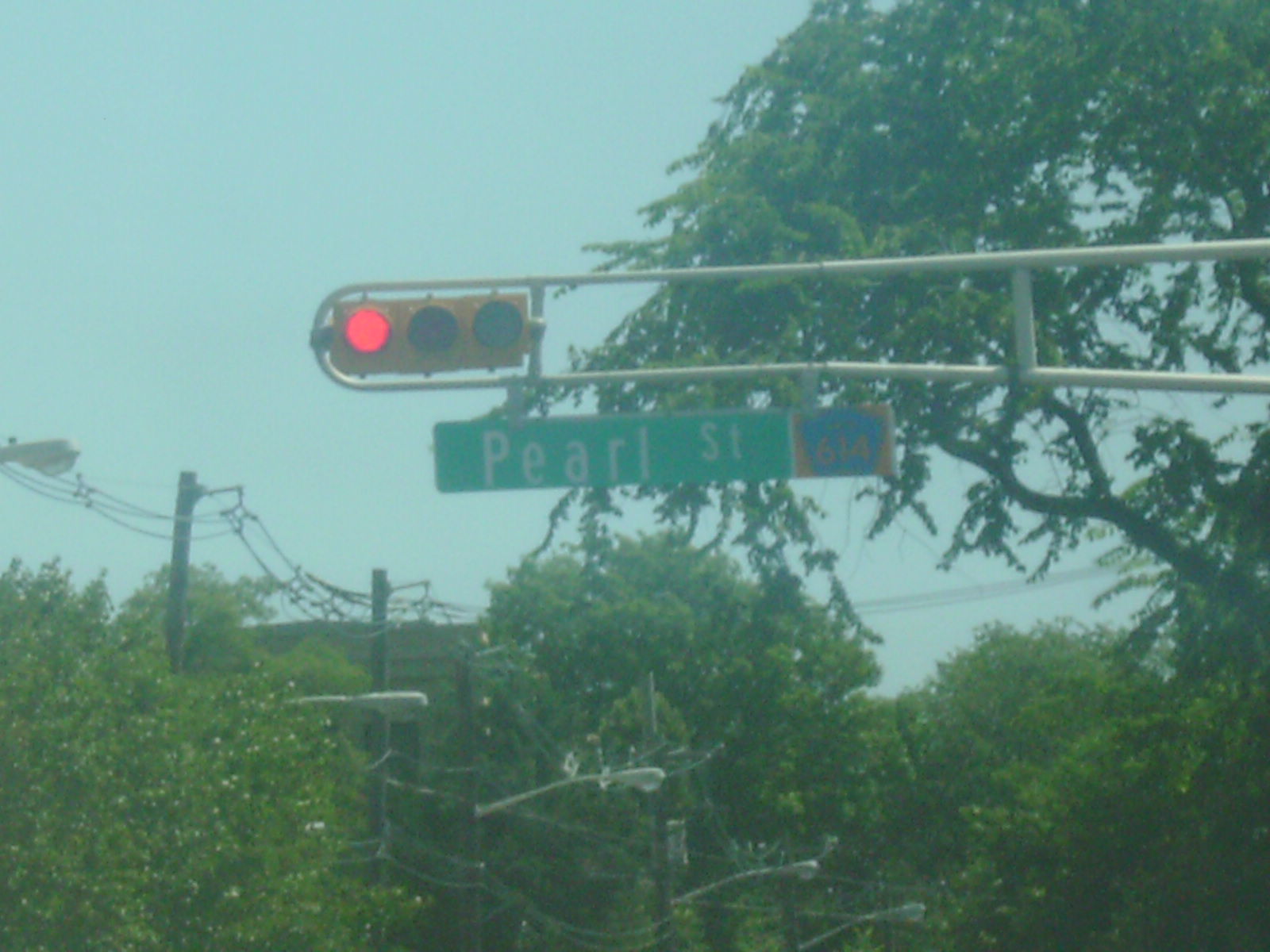The image captures an outdoor setting with a medium blue, slightly hazy sky overhead, devoid of any visible clouds. It's a daytime scene in either a city or suburban area, as suggested by the presence of multiple tall trees, telephone poles, and streetlight fixtures. Dominating the foreground is a towering tree with a modern horizontal traffic signal suspended in front of it. This traffic signal is affixed to two extended metal rods, with the red light illuminated, indicating a stop. Just below the traffic light, a green street sign with white lettering announces "Pearl Street." The photograph appears to be taken from a lower angle, providing a high-up perspective that accentuates the verticality of the scene. To the left side of the image, telephone lines crisscross through the frame, while the tops of streetlights, switched off in the daylight, can be seen further down the street on the opposite side. The overall atmosphere is calm, encapsulating a typical moment in an urban or suburban locale.